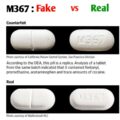Caption: The image is a detailed reference guide designed to help identify the difference between a fake and a real pill labeled "M367." The guide is clearly titled "M367: Fake vs. Real" with the words "Fake" highlighted in red and "Real" in green, while "vs." is also in red. The guide features two side-by-side pictures of pills on a white background. Each picture contains two white pills; on the left is a white capsule, and on the right is a white tablet. The tablet notably bears engraved characters that seem to spell out "M367." Between the two pictures, there is a block of black text, though it is blurry and difficult to read. This guide aims to provide a visual comparison to aid in distinguishing authentic medication from counterfeit versions.